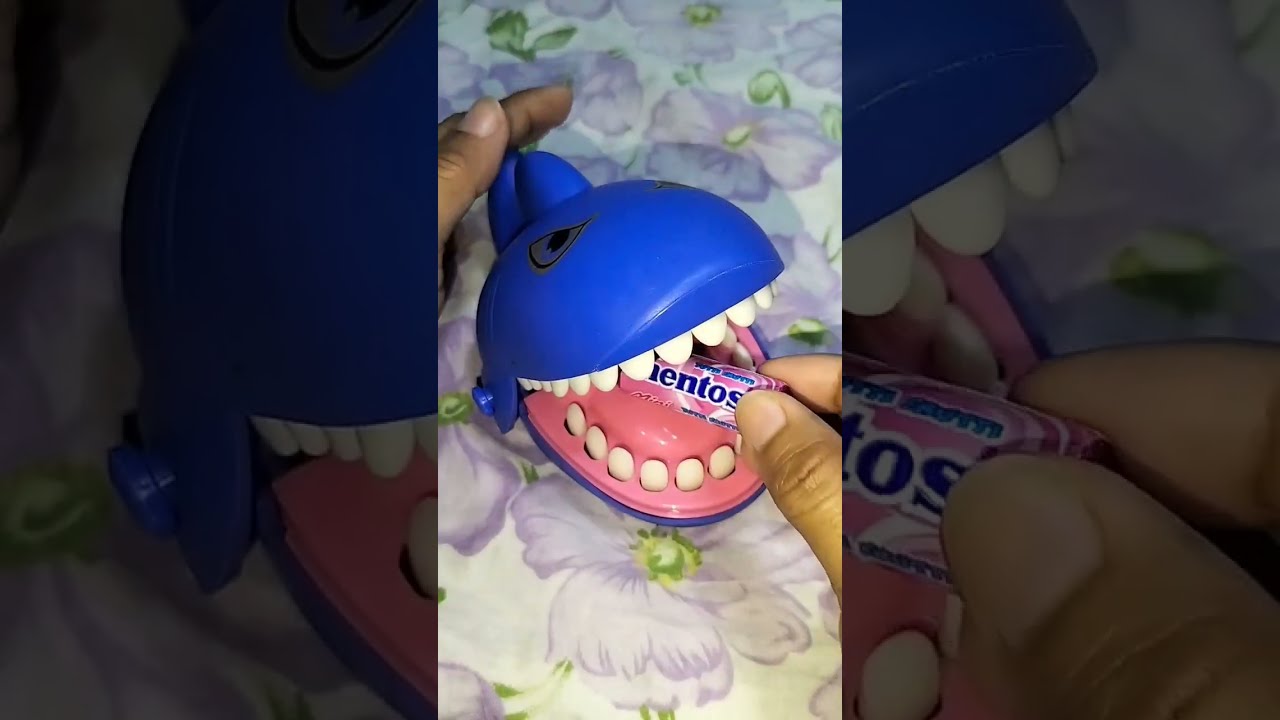In the image, a captivating composition is formed by three panels, with the central panel brightly illuminated and the side panels darkened to draw focus. The central panel presents an intriguing close-up of a blue toy shark, its giant pink mouth lined with large white teeth open wide. The shark, with visible eyes atop its head, appears vivid against a backdrop of a vinyl tablecloth adorned with a purple and white floral pattern accompanied by green leaves. Two dark-skinned hands with short, unpolished nails are positioned on either side of the image. The left hand grasps the toy shark, positioning its mouth akin to a Pez dispenser, while the right hand holds a round package of Mentos candy, distinguished by its primarily pink wrapper with "Mentos" inscribed in bold dark blue letters on a white border. The Mentos tube is seen halfway into the shark's gaping mouth, creating a whimsical juxtaposition. The side panels subtly frame this playful scene, emphasizing the details and bringing full attention to the vibrant and detailed main depiction.